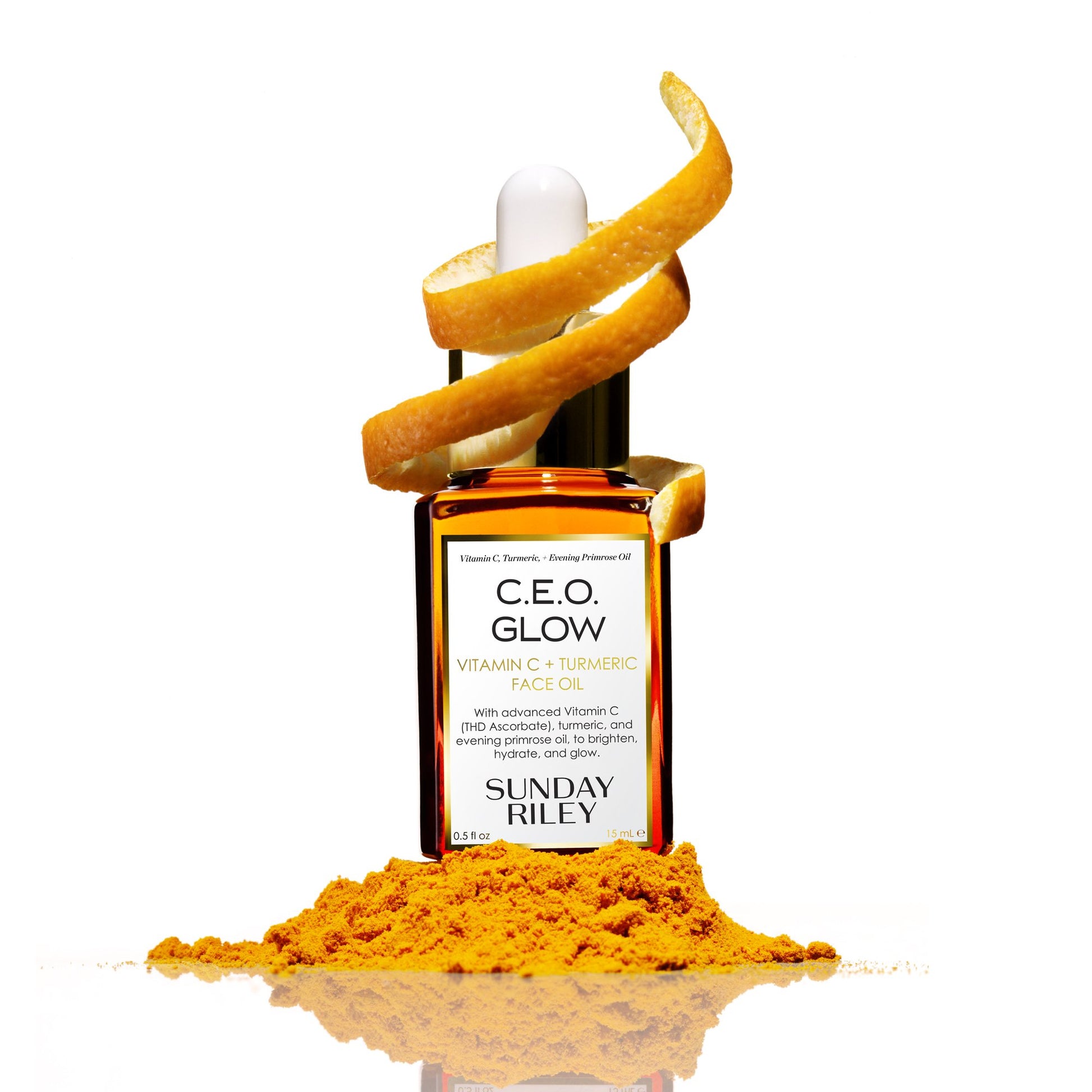The image showcases an advertisement for Sunday Riley's C.E.O. Glow Vitamin C + Turmeric Face Oil. Set against a plain white background, the focus is on a small, square, clear glass bottle containing an amber-gold liquid. The bottle has a gold cap with a white rubber dropper attached, and an orange rind elegantly wraps around the top. The front label reads "C.E.O. Glow" in prominent black text with details including "Vitamin C + Turmeric Face Oil with Advanced Vitamin C, THD Ascorbate, Turmeric, and Evening Primrose Oil to brighten, hydrate, and glow." Below the product name, it indicates the size, 0.5 fluid ounces (15 mL). There’s a reflection effect beneath the bottle, accentuating a small pile of orange turmeric powder positioned at the base, enhancing the vibrant and health-oriented theme of the product.